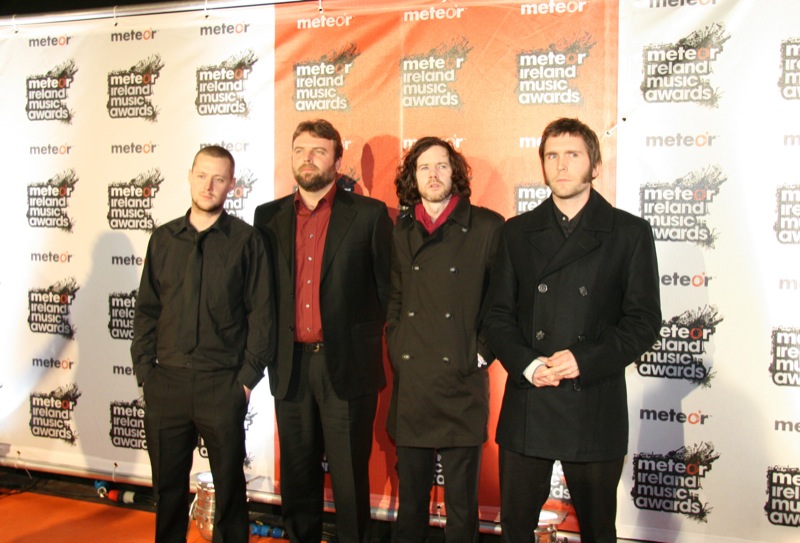The image captures a photograph of four men standing in front of a promotional banner wall for the Meteor Ireland Music Awards. The banner has a repeating logo with text that reads "Meteor Ireland Music Awards" in white font outlined in black, and features a fiery, splotchy illustration in brown and red that appears to represent a falling meteor.

From left to right, starting with the first man who is visible only from his ankles upwards, he is dressed in black pants and a long-sleeved button-up shirt with a black tie. His collar button is undone. Next to him is a man wearing black pants with a belt, a red button-up shirt with the collar also undone, and a black business coat. The third man stands out with his gray business pants and a front double-breasted jacket, accompanied by a red shirt underneath. Finally, the fourth man is seen wearing both a black coat and black pants.

The men display various expressions, ranging from neutral to slightly bored. The photograph distinctly highlights their different styles and attire against the backdrop of the event's vibrant and repetitive logo design.